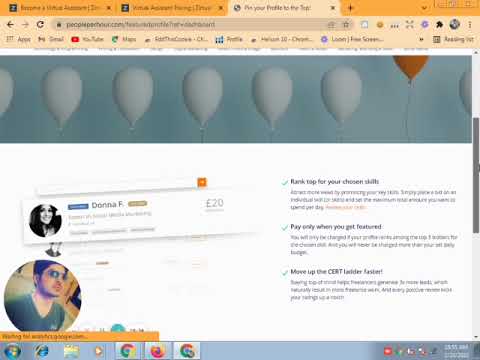In this detailed screenshot taken from a Windows computer, the central focus is on a Google Chrome tab displaying a website, with an almost full-screen view. The desktop's familiar start menu and browsing icons are visible at the bottom, indicating it’s indeed a Windows OS. The top portion of the website features a dull blue background adorned with several balloons, predominantly light blue and gray, but with a distinctive dark mustard-colored balloon that is partially cut off as it floats upward. 

The site appears to begin with the letter 'P' and contains an illegible URL due to the blurriness. The text on the page is mostly unreadable, though there are snippets such as "Donna F. Rank top for your chosen staff" and "Pay only when you get featured." Visual elements also include two small photos in the bottom left corner—a larger image of a male wearing glasses and a dark blue V-neck shirt, and a smaller image of a woman. These photos are accompanied by a range of colors throughout the screenshot, including orange, light peach, yellow, red, light blue, green, and gray. Overall, the image style suggests a digitally created or software application environment.